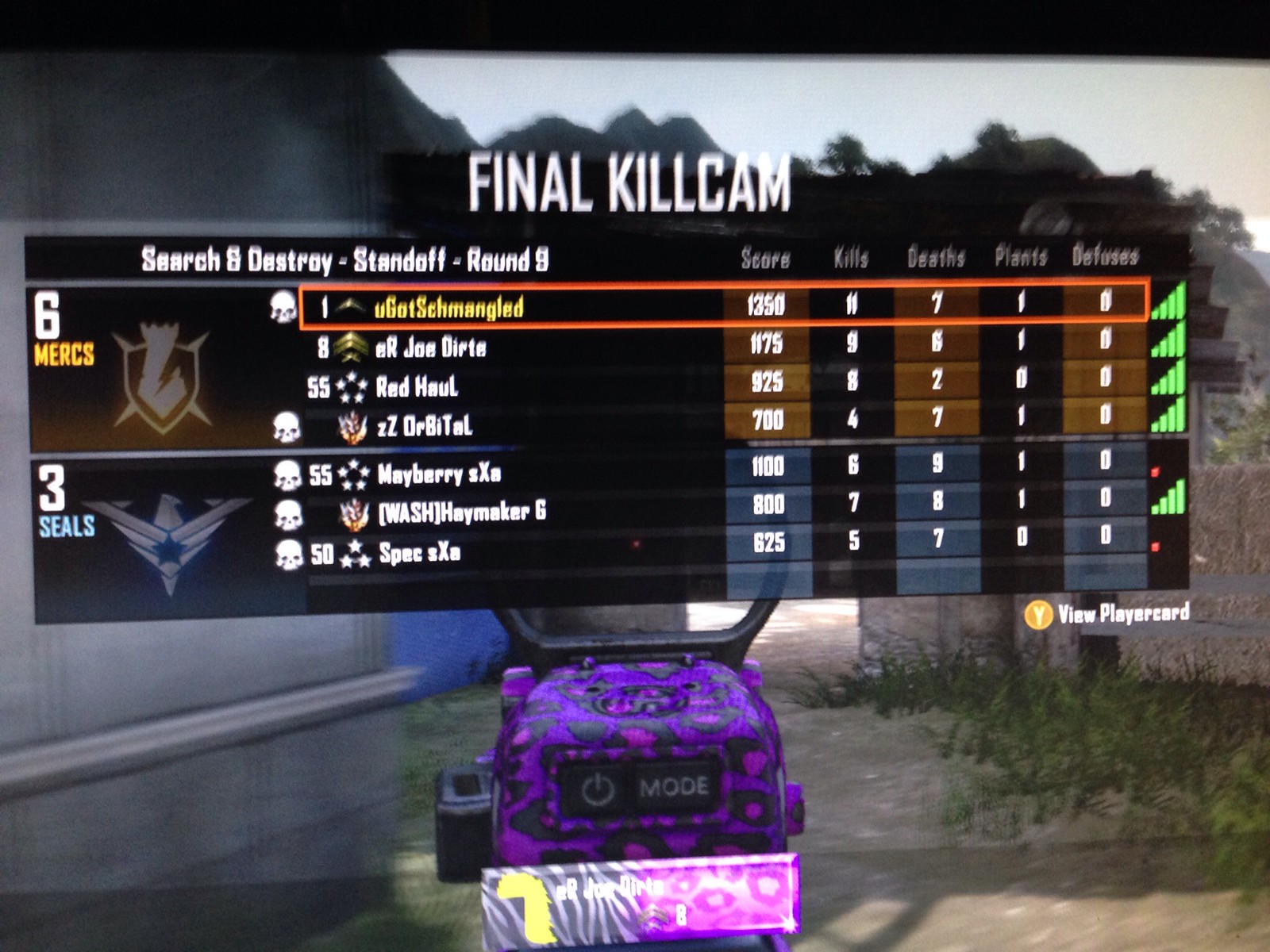The image is a clear screenshot from the video game Call of Duty, displaying its Final Kill Cam. At the top, it reads in all capitals "FINAL KILL CAM," "Search and Destroy," "Standoff," and "Round 5." It shows a duel between two teams: the Mercs leading with a score of 6 and the Seals trailing at 3. The screen also details individual player statistics, including kills, deaths, plants, and defenses, accompanied by team logos—an Armored Soldier of Arms for the Mercs and what appears to be a jet for the Seals. The center of the screen prominently displays a vibrant purple and pink gun, complete with zebra and cheetah patterns, aiming down its scope. The gun features a button labeled "Mode." Additionally, the bottom of the screen shows a yellow circle with a "Y," instructing players to view the player card. This well-lit image captures the intensity and detailed design of the gameplay environment.